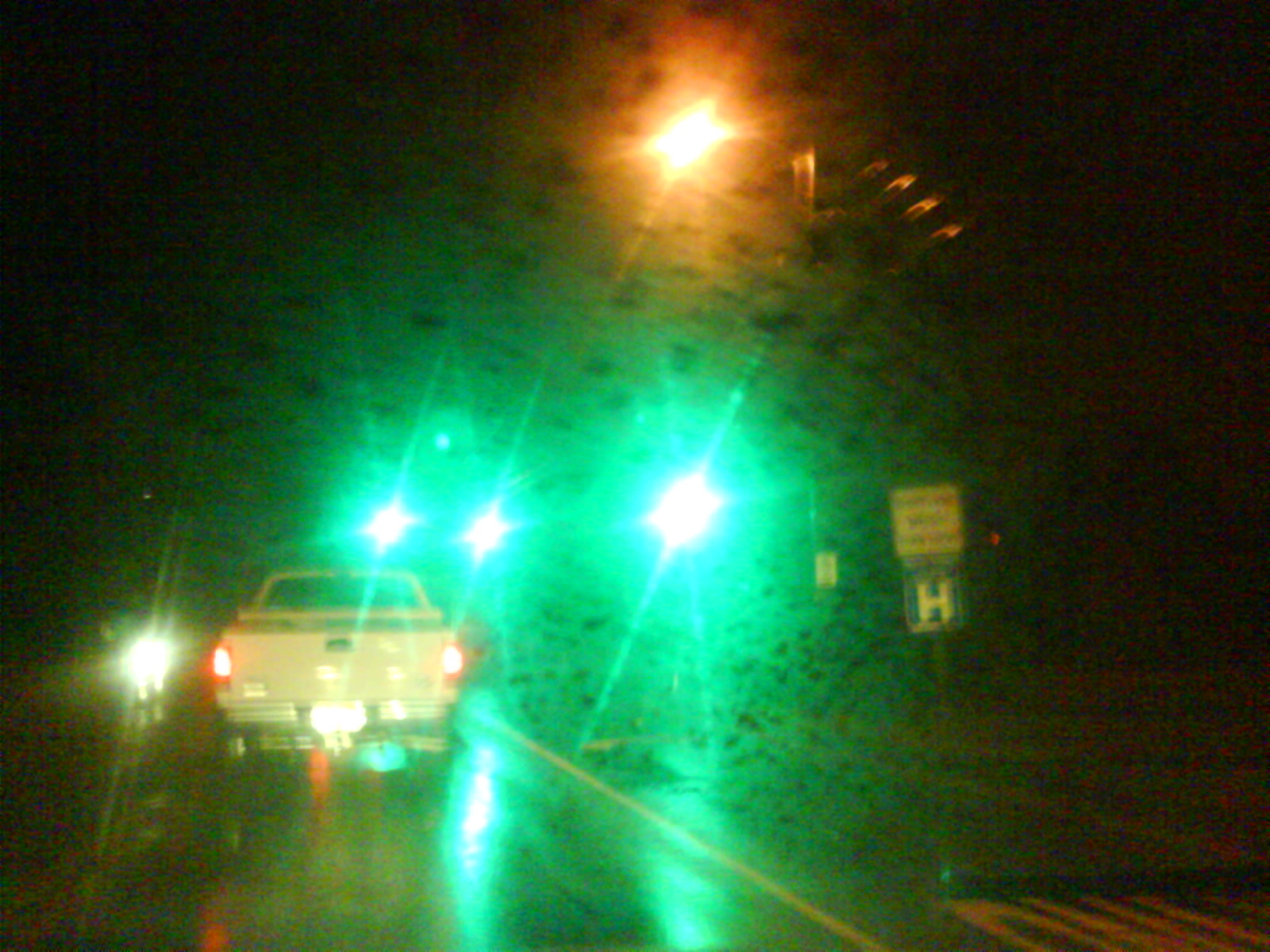A blurry nighttime photograph taken from the dashboard of a moving vehicle captures the scene ahead. Dominating the foreground is a white pickup truck with its red rear taillights illuminated. Further down the road, a circular white light is visible, with a few additional distant lights floating just above it. A street lamp on the right side casts a yellowish glow, surrounded by an orangey halo that contrasts with the darkness. Near the street lamp, a roadside sign comes into view: a square with a white "H" at its center, topped by another square sign in white with some unreadable text. The white lines marking the outer lane of the road add subtle definition to the otherwise diffuse image.